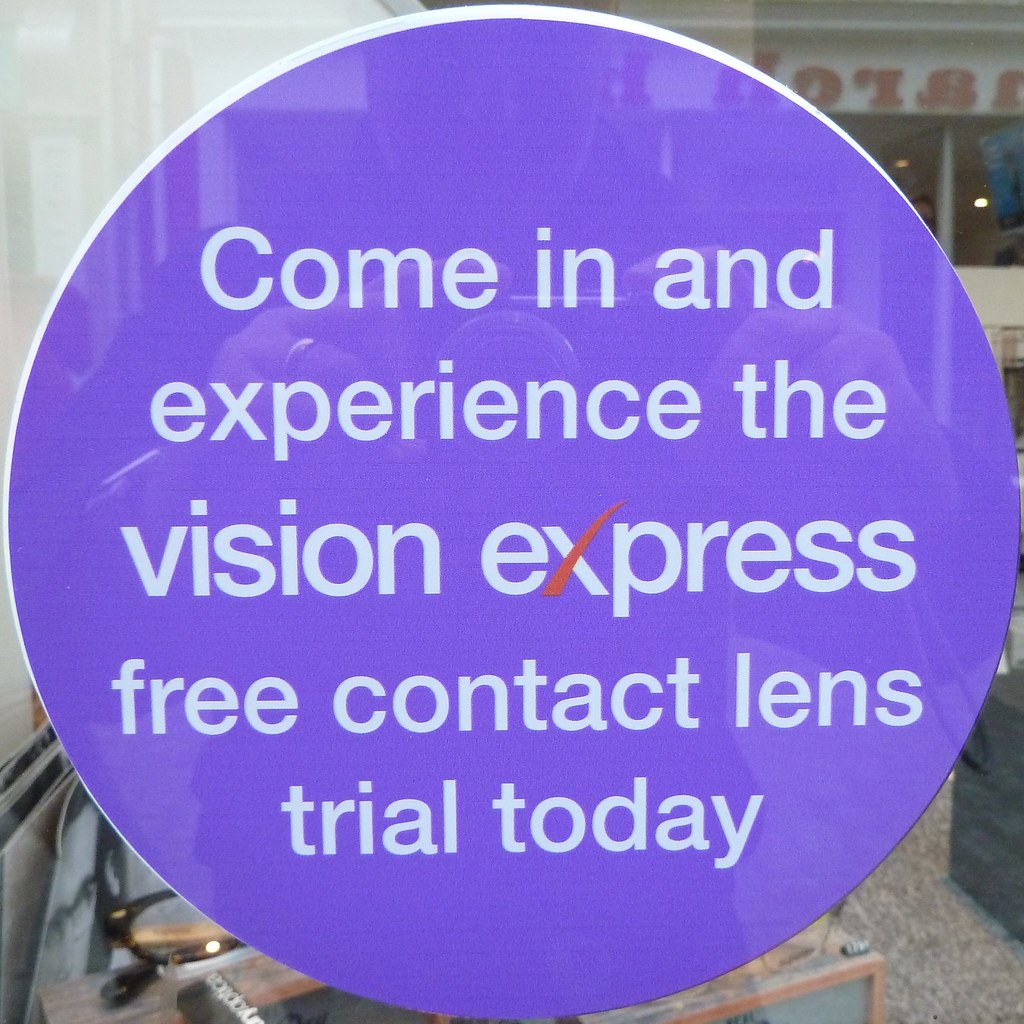This photograph captures a circular promotional sign adhered to the glass window of a retail optometrist's office called Vision Express. The sign features a purple background with white text that reads, "Come in and experience the Vision Express free contact lens trial today," with the "X" in "Express" notably styled with one red and one white line. Taken through the glass, the image reveals reflections of the photographer, who is close enough that their ring is visible; reflections also include a store located across the street. Inside the establishment, partial views of a table and chair can be discerned, suggesting a welcoming lobby or reception area typical of an optometrist's practice.